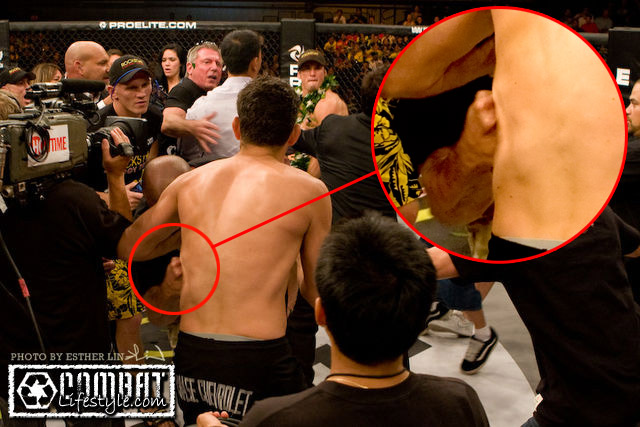The photograph captures a dynamic moment featuring multiple MMA fighters in an octagon. At the center of the image is a shirtless man facing away, wearing black pants with a gray waistband peeking out from underneath. On closer inspection, indicated by a circle and a line pointing to a zoomed-in section of the image, another fighter is shown landing a punch to the ribs of the shirtless man. Surrounding them are several individuals, including a cameraman with a 'Showtime' logo on his black shirt, capturing the scene. The background showcases a chain-link fence typical of MMA rings, with 'ProElite.com' inscribed in white letters at the top. In the bottom left-hand corner, there's a watermark that reads 'Photo by Esther Lin' and 'CombatLifestyle.com' inside a white rectangle. The scene appears to be post-match, indicated by the presence of multiple people and media equipment around the fighters.